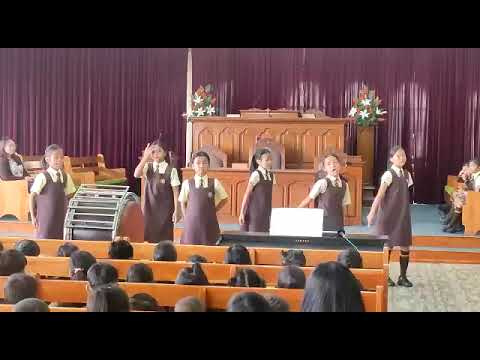The image appears to be a blurry screen capture from a video, characterized by black horizontal bars at the top and bottom. It depicts a scene inside a church, specifically focused on the altar area adorned with light brown wooden elements and podiums with flowers on either side. The backdrop is a maroon-colored curtain extending from the ceiling to the floor.

At the center of the image, six young girls, likely around 9 to 10 years old, stand in a uniform line. They are dressed uniformly in white short-sleeved shirts with brown dresses over them, complete with ties, pull-up brown socks, and shoes. All the girls have dark black hair pulled back into ponytails and appear to have light brown skin. They seem to be performing—perhaps singing—given the presence of a large drum and at least one girl appearing to sing.

The foreground features at least four rows of wooden pews, predominantly occupied by children, with only their heads visible above the seat backs, indicating they are quite small in stature. A few adults can also be spotted among them. Additionally, more pews are visible on either side of the image: some on the right side lined with other girls, possibly waiting for their turn, and others on the left side, including a woman seated in a bench.

The communal setting and the coordinated attire of the girls suggest this is likely a school performance taking place in a church, with the children in the congregation attentively watching their peers on stage.